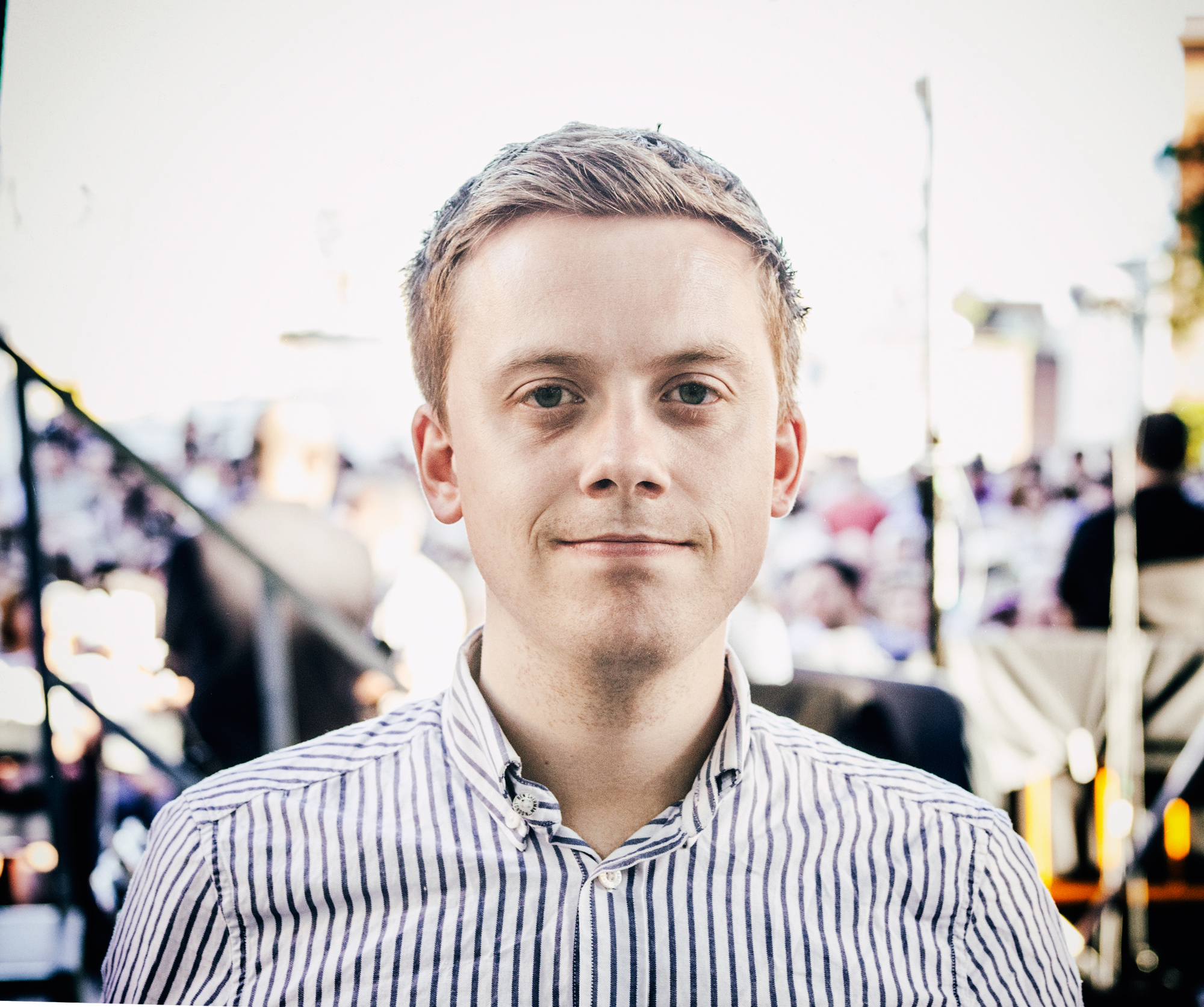The photograph captures a young man, possibly in his twenties or early thirties, seen from his upper chest to the top of his head. He has very short blonde hair, swept back, and light brown eyebrows. His captivating gray-blue eyes and semi-smirk give him a subtle, approachable demeanor. He wears a white button-up shirt adorned with vertical blue stripes, with the top collar button stylishly undone and clear acrylic buttons down the front. Both sides of his collar are buttoned down. The background behind him is heavily blurred, revealing an indistinct group of seated people, suggesting a possible event or gathering. The focus remains on the man, highlighting his composed yet slightly smiling expression against the obscure crowd.